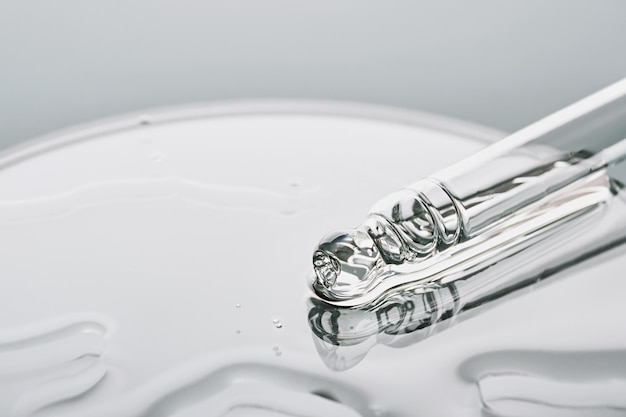The image depicts a close-up scene with a glass eyedropper depositing liquid onto a reflective surface, which appears to be a petri dish or a clear plastic platform. The gray background wall makes the details slightly harder to distinguish. The eyedropper, entering the frame from the right-hand side, shows small air bubbles near its tip, highlighting the liquid's movement. The reflective surface beneath the dropper has liquid spillage, reflecting the transparency and clarity of the eyedropper and enhancing the shiny, swirling design of the cylindrical tool. The overall picture is in black and white with varying shades of light gray, enhancing the contrast between the reflective surface, the clear eyedropper, and the plain gray background. The surface has visible grooves, including a partial V-shaped groove in the middle, adding to the intricate details of the image.